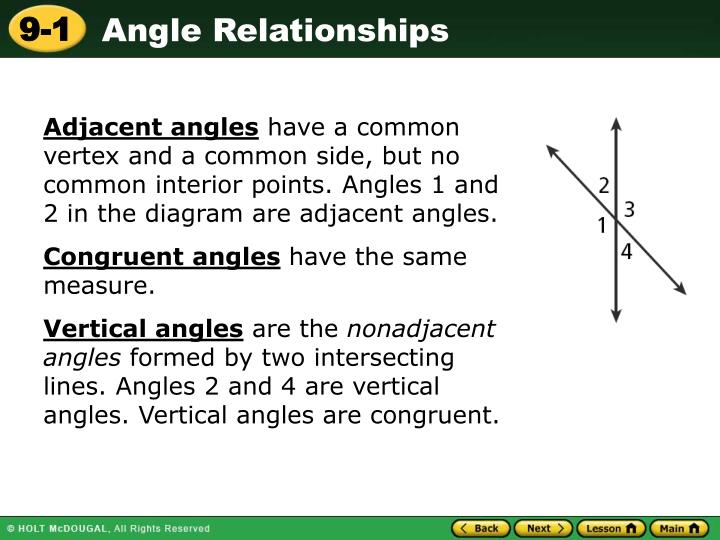The image appears to be a screenshot of an educational website on the topic of angle relationships from Holt McDougall. The slide is titled "Angle Relationships" in white text on a green background at the top, and indicates it's for Chapter 9-1 with the chapter number "9-1" displayed in black text on a yellow oval in the upper left corner. The left side of the image contains three small paragraphs, each with a bold underlined heading:

1. **Adjacent Angles:** Describes that adjacent angles have a common vertex and a common side but no common interior points, exemplified by angles 1 and 2 in the diagram.
2. **Congruent Angles:** States that congruent angles have the same measure.
3. **Vertical Angles:** Explains that vertical angles are the non-adjacent angles formed by two intersecting lines, with angles 2 and 4 given as an example of vertical angles, noting that vertical angles are congruent.

The right side of the image features a diagram showing two intersecting lines. One line is vertical while the other has a steep negative slope, creating four angles labeled clockwise from the bottom left as 1, 2, 3, and 4. 

At the bottom of the slide, a green bar includes a copyright notice stating "Holt McDougall, all rights reserved." On the far right side, there are yellow navigation buttons with black text labeled "Back," "Next," "Lesson," and "Main," each accompanied by relevant icons.